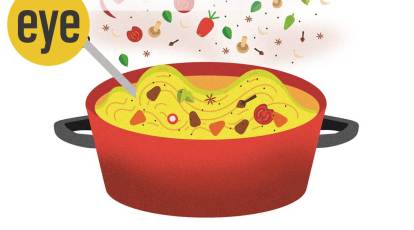The image is a cartoon illustration of a bright red cooking pot, which transitions to a darker red at the bottom. It has flat sides and a circular shape with two dark gray circular handles on each side. The interior is also red at the lip, with a bright yellow substance inside that looks like wavy, yellow soup or noodles. Scattered within the soup are various colorful items, including red, orange, green, and brown pieces, some of which resemble vegetables like tomatoes, onions, mushrooms, peppers, and possibly radishes. There are also star shapes, small black circles, a strawberry, and other small geometric shapes in orange, white, and brown. Above the pot, additional food items appear to be falling in, such as tomatoes, an apple, green leaves, and more. In the upper left corner of the image, a yellow circle contains the word "eye" written in lowercase black letters, with a gray bar or arrow extending down from it into the pot.